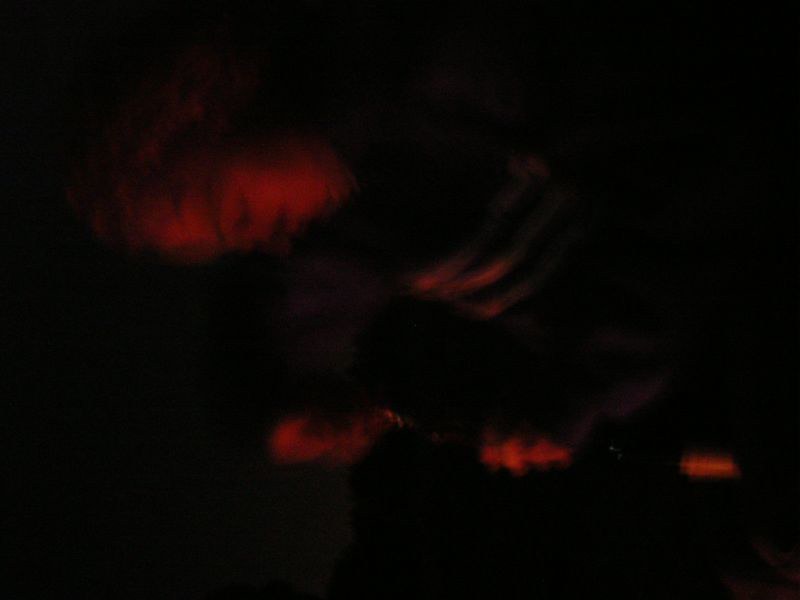In this photograph, a spectral figure is captured in a hauntingly dark and disorienting frame. The image, turned on its side, portrays what appears to be a ghostly woman, though the gender is indistinct due to the blur. She is seated on a sofa chair, but the sideways orientation makes her body seem to be facing downward. The most striking element is her face, which is bathed in an eerie red glow from an unidentified light source, adding to the otherworldly effect. She wears a shirt adorned with three white stripes, though the color of the garment remains indiscernible. In her left hand, she clutches a short staff, highlighted faintly by the same mysterious red light. The overall photograph is engulfed in pitch-black darkness, with only the glowing face and the staff piercing through the gloom, further emphasizing the unsettling, ghostly ambiance.